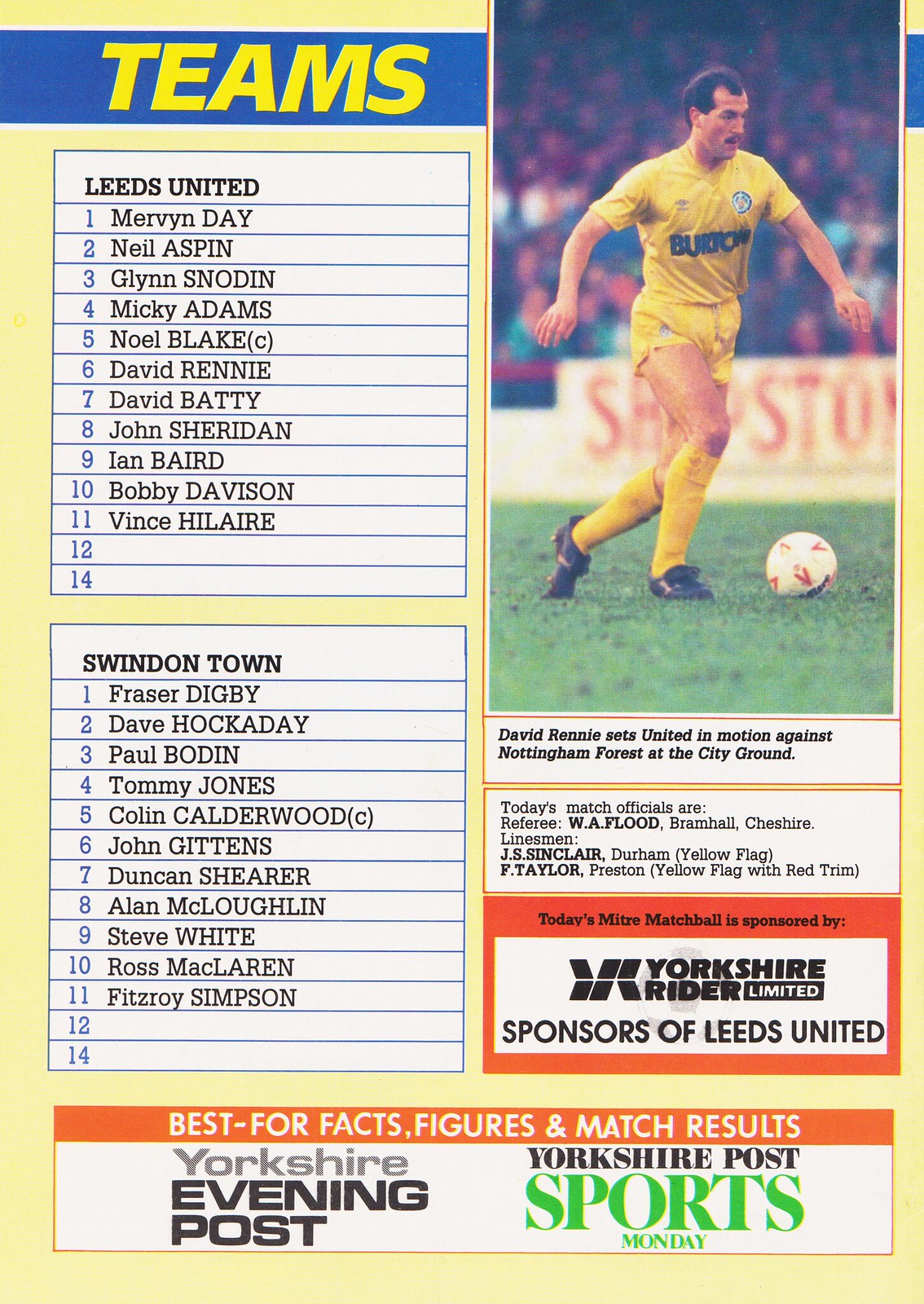The rectangular image appears as a comprehensive page from a sports program or magazine. Dominated by vibrant colors, it features a photograph in the top right corner showing a soccer player on the field mid-kick. The player, donned in a complete yellow kit—with a yellow jersey, shorts, and tall socks paired with black cleats—is captured against a backdrop of blurred fans in the stadium. The top left corner of the page highlights a blue banner with the word "Teams" boldly printed in yellow. Below this, two detailed rosters for Leeds United and Swindon Town are listed, each featuring player names numbered from 1 to 11. Adjacent to the photograph, a caption reads, "David Rennie sets United in motion against Nottingham Forest at City Ground." Further down, another box specifies the match officials, including the referee, W.A. Flood, and linesmen, J. Singler, and F. Taylor. Below the officials’ details, a sponsor advertisement for Yorkshire Rider Limited acknowledges their support of Leeds United with a red-bordered box. Finally, the bottom of the page is accented with an orange banner announcing "Best for facts, figures, and match results," flanked by the logos for Yorkshire Evening Post and Yorkshire Post Sports Monday.